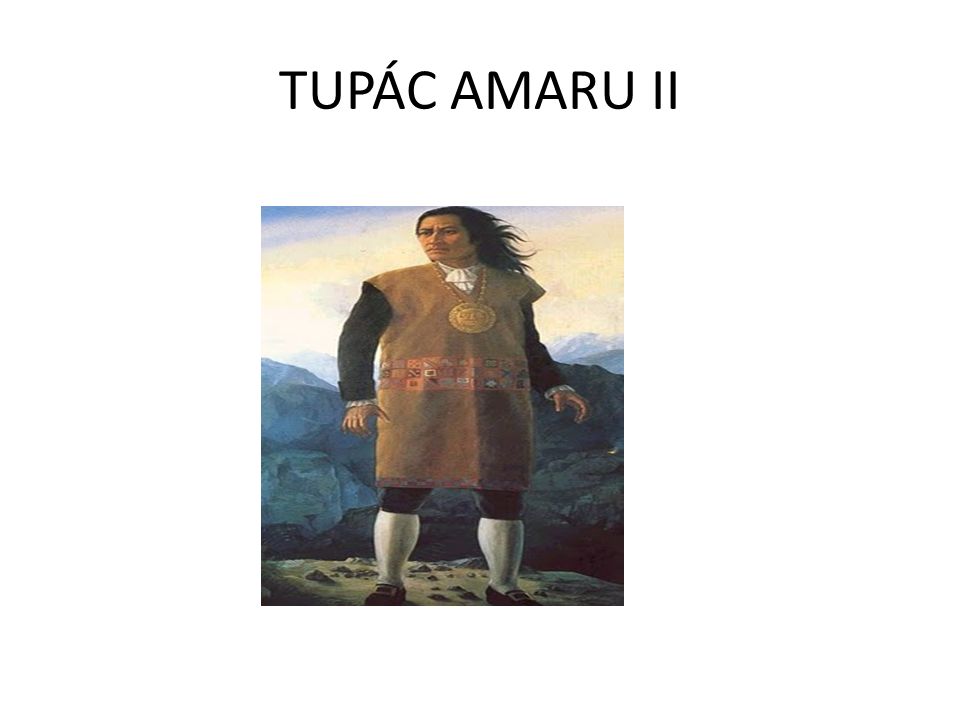This detailed illustration depicts Tupac Amaru II, with his name inscribed in black lettering at the top. He stands in a noble posture against a backdrop of gray mountains and a cloudy white-blue sky. His long, flowing black hair is swept back by the wind as he gazes resolutely to the left. Dressed in a striking brown tunic decorated with multicolored accents over a red base, he dons black sleeves paired with black pants and white stockings that reach his knees, accentuated by black shoes with buckles. Central to his attire, a large golden medal shines on his chest above a white cravat. The painting captures him alone, seemingly on the crest of a hill, conveying a sense of solitary defiance and grandeur.